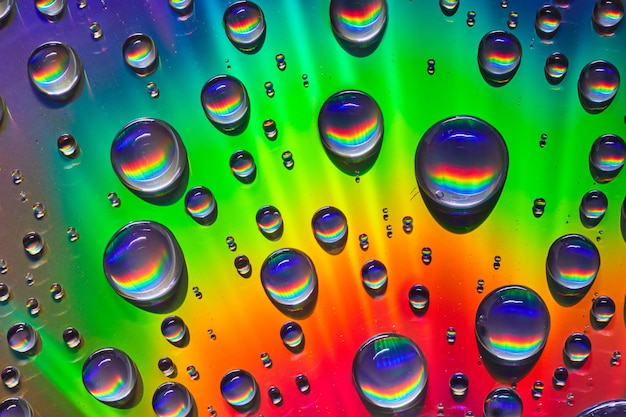This image depicts an incredibly detailed and vividly colorful scene, likely computer-generated or heavily photoshopped. The background features a gradient rainbow burst effect transitioning from red in the bottom right to orange, yellow, green, teal, blue, and finally violet at the upper left. Bright rays of yellow and other colors streak through this vibrant backdrop. Scattered across this radiant surface are approximately 50 to 100 water droplets of varying sizes, ranging from large to small spheres and hemispheres. These droplets reflect a rainbow pattern within themselves, though it does not seem to match the rainbow gradient on which they rest. The larger drops distinctly show this internal rainbow, while the smaller ones reflect it more subtly. Each droplet casts a shadow below, indicating a light source from above, enhancing their three-dimensional appearance and volume. The scene is richly colorful and captivating, with each droplet and ray contributing to the overall impression of a fantastical, surreal landscape.